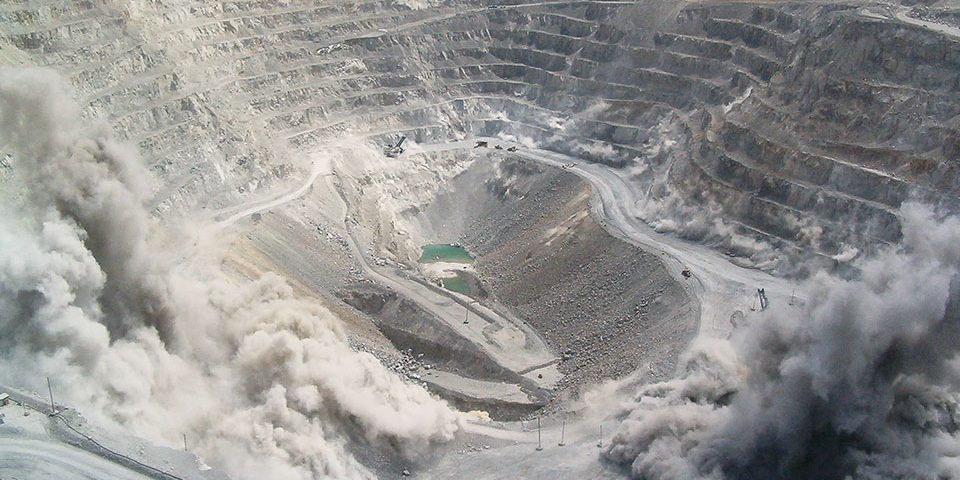The landscape-oriented image captures a distant view of a deep and expansive operational quarry. The quarry stretches hundreds of yards both in depth and breadth, with a striking theater-like arrangement of terraces cascading upward and outward from a central pit. At the very bottom of the pit lies a greenish aquamarine body of water, likely formed from rain runoff. The area is enveloped in thick clouds of dust, stirred up either by the activities of vehicles or by the wind. Above and beyond the central water body, faint outlines of machinery—such as cranes and large trucks—can be observed, indicating ongoing mining operations. One side of the image is particularly hazy, shrouded in dust or possibly fog, and features what seems to be a partially collapsed road, adding to the scene's rugged and active atmosphere. Despite the overall clarity, the haze and machinery contribute to a sense of intense industrial activity within this immense, meticulously tiered excavation site.